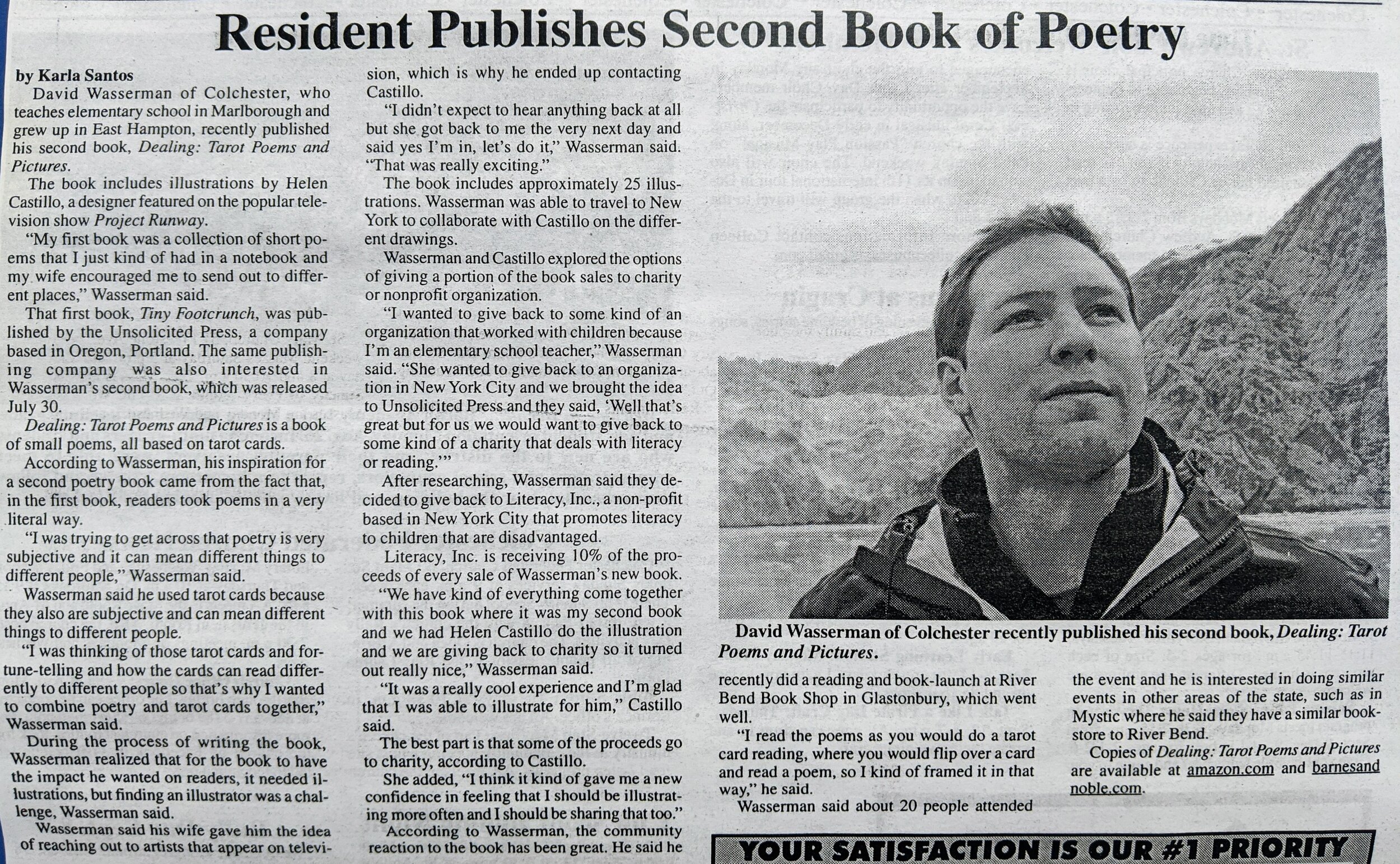"Black-and-white newspaper clipping showcasing a headline in a bold, 20-point font, 'Resident Publishes Second Book of Poetry.' Below the headline, author details are prominently displayed: 'by Carlos Santos,' misspelled as 'K-A-R-L-A Santos.' The left-hand side of the page features two columns of text, with the first paragraph highlighting David Wasserman of Colchester, an elementary school teacher in Marlborough who grew up in East Hampton, and his recent publication, 'Dealing, Tarot Poems and Pictures.' The text also mentions the book's illuminations by Helen Castillo, a designer famed for her appearance on Project Runway. The right-hand side is dominated by a photograph occupying 80% of the space, depicting David Wasserman hiking in the mountains, gazing towards the sky. Below the image, a brief caption reiterates the publication details: 'David Wasserman of Colchester recently published his second book, Dealing, Tarot Poems and Pictures.' At the very bottom, partially cut off, an advertisement snippet reads: 'your satisfaction is our number one priority,' adding a commercial touch to the otherwise literary-focused article. The entire layout, from text to imagery, is captured in monochrome, emphasizing the vintage newspaper aesthetics."